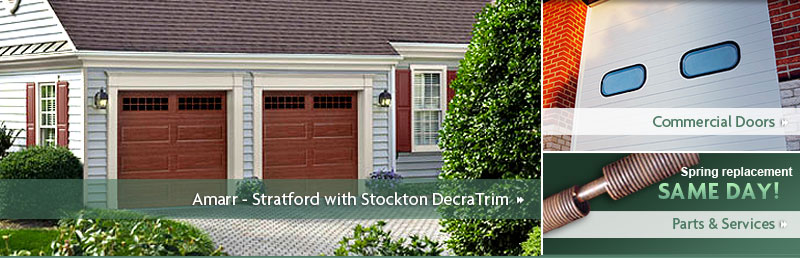**Advertisement Caption:**

The advertisement features three distinct photographs and a central, long rectangular promotional message. On the left, there is an image of a charming single-family house with gray siding and tan-brown garage doors beneath a stylish slate roof. The home is accentuated with well-maintained landscaping and bushes, establishing an inviting curb appeal. Below this image, the text reads: "Amar Stratford with Stockton Decoratrim."

To the right, the upper photograph highlights a large commercial white door adorned with two oval windows, set against a brick exterior. The caption above this image states: "Commercial Doors." 

Beneath it, another image shows a rusted garage door spring along with the text: "Spring Replacement - Same-Day Parts and Services." 

The background of the advertisement is a vibrant green, adorned with white and green lettering. Thin white lines neatly separate each image, adding to the clean and organized layout of the advertisement.